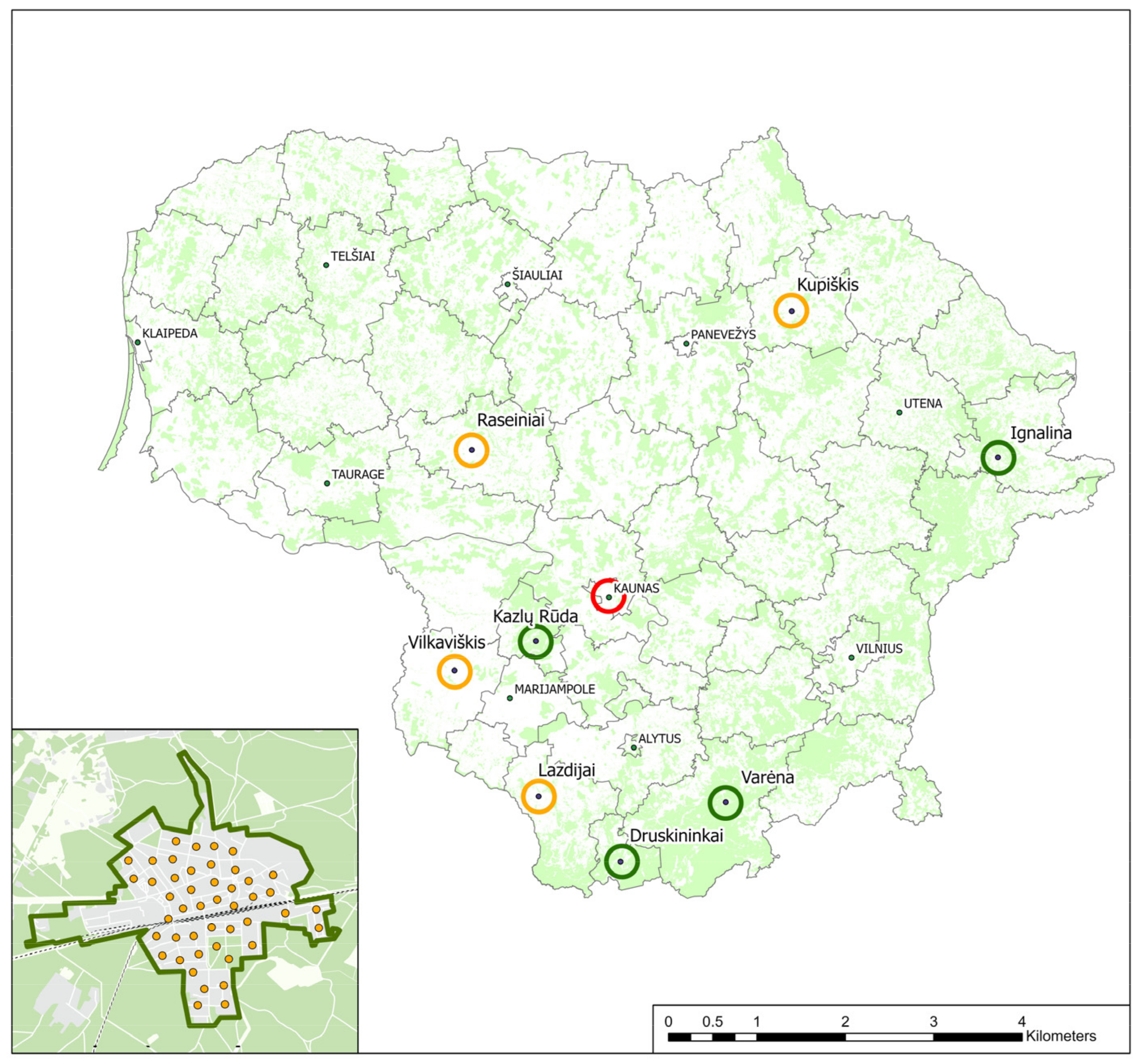This is an intricate, hand-drawn topographical map, likely of a country or continent, featuring various geographical and urban details. The map consists of numerous regions delineated in muted dark gray, with shading in different tones of green and white. Darker green areas suggest higher population densities, while lighter green and white areas indicate less populated or possibly forested regions. Key locations, presumably cities, are marked with a combination of green dots, yellow circles, and red circular dots. Some of the labeled cities include Ignalina, Kupiskis, Kelpia, Telsia, Siatra, Penezuelas, Penesacas, Resalanti, Drugon, Villacancias, Casirruda, Marriapul, Las Jutas, Alturas, Dronitzky, Berina, Villaness, Galena, Utenia, and Canunas. A standout feature is the red-circled city of Kalinas, which may be a capital or a significant urban center. There is an inset map that offers a close-up view of one of these cities, bordered in solid green and dotted with orange circles, although it lacks a legend explaining these details. The left-hand side of the map includes an aerial legend, while the bottom right features a distance scale in kilometers, providing a practical tool for measuring distances across regions, indicative of the map's non-U.S. origin.